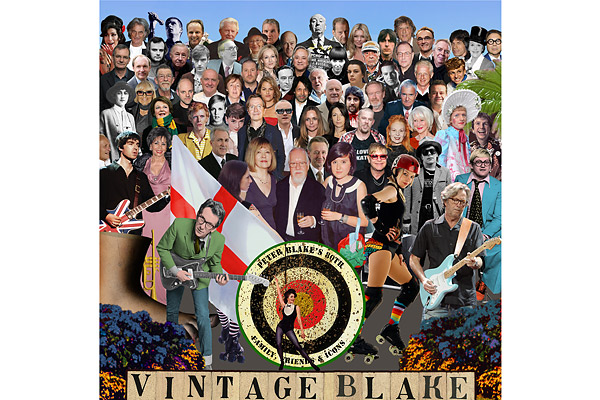The image appears to be a vibrant, square artwork resembling a vinyl album cover, designed in a collage style reminiscent of Peter Blake's iconic pieces. At the bottom of the cover, the phrase "Vintage Blake" is prominently displayed in block letters, which are light brown with black text. Just above this, there is a prominent bullseye design featuring yellow, red, and black concentric circles. Inside the bullseye, text reads "Peter Blake’s Family, Friends and Icons." The artwork is a rich tapestry of various cut-out images of people, some recognizable and others less so. Among the celebrities featured are iconic figures such as Elton John, Alfred Hitchcock, Buddy Holly playing a guitar on the left, and Eric Clapton holding a blue electric guitar on the right. Additionally, there is a woman on roller skates and a figure in a green suit jacket playing an electric guitar. The composition also includes colorful flowers positioned in the bottom left and right corners, further enhancing the collage’s eclectic and nostalgic feel. The entire piece evokes a sense of homage to Blake's classic style, similar to the famous "Sgt. Pepper's Lonely Hearts Club Band" album cover.